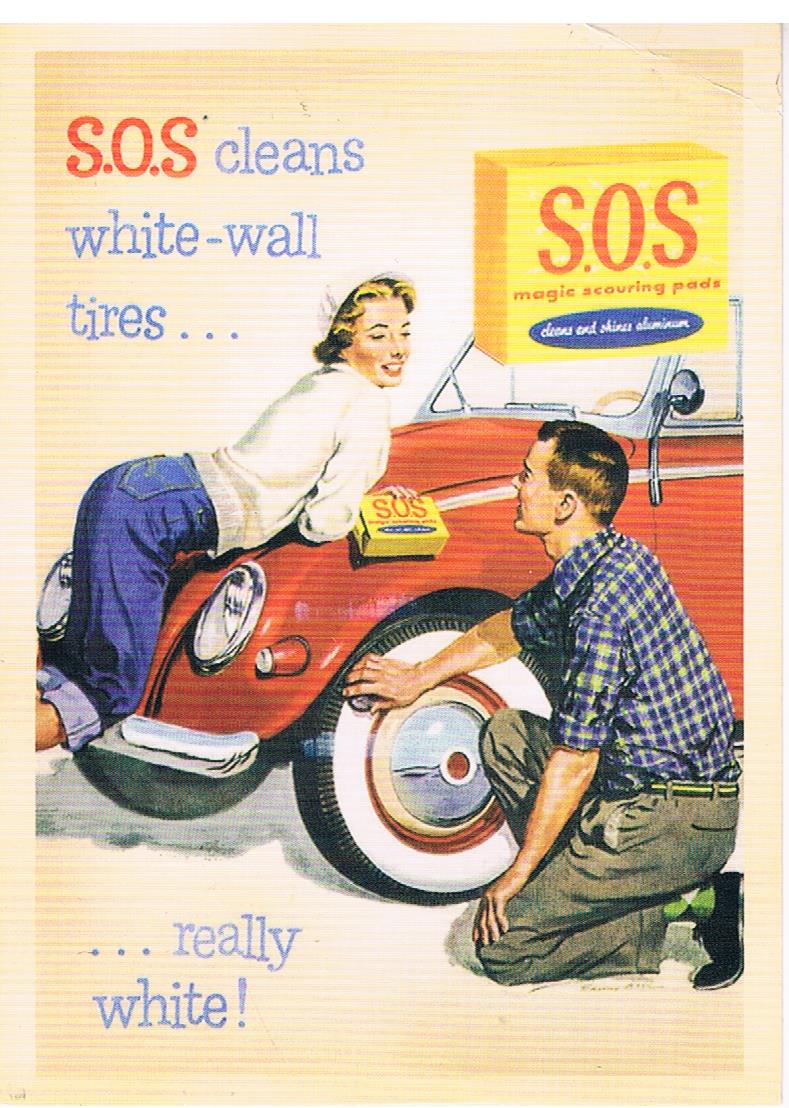The image depicts a vibrant, old-fashioned advertisement in comic-style art for SOS Cleaners, appearing on what looks like a magazine or perhaps a sign. The background is yellow, enhancing the bright and clear visual appeal of the artwork. Central to the scene is a woman leaning against the front bumper of a red Volkswagen, holding a yellow box of SOS scouring pads, with the "SOS" prominent in red text. She is dressed in a plaid blue and green shirt paired with brown trousers. In some descriptions, she is alternatively noted to be wearing a white sweater and blue jeans cuffed at the bottom. Adjacent to her, a man is on one knee, diligently scrubbing the white wall of the tire. He is depicted wearing a blue flannel shirt and green pants, occasionally described as brown trousers. Text across the image emphasizes the cleaning power of the product with slogans such as "SOS cleans white wall tires" and "SOS magic scouring pads" at the top. Additionally, a noteworthy detail in the bottom left corner exclaims "Really white!" The overall scene is colorful, nostalgic, and clearly promotes the effectiveness of SOS scouring pads in providing sparkling clean white wall tires.